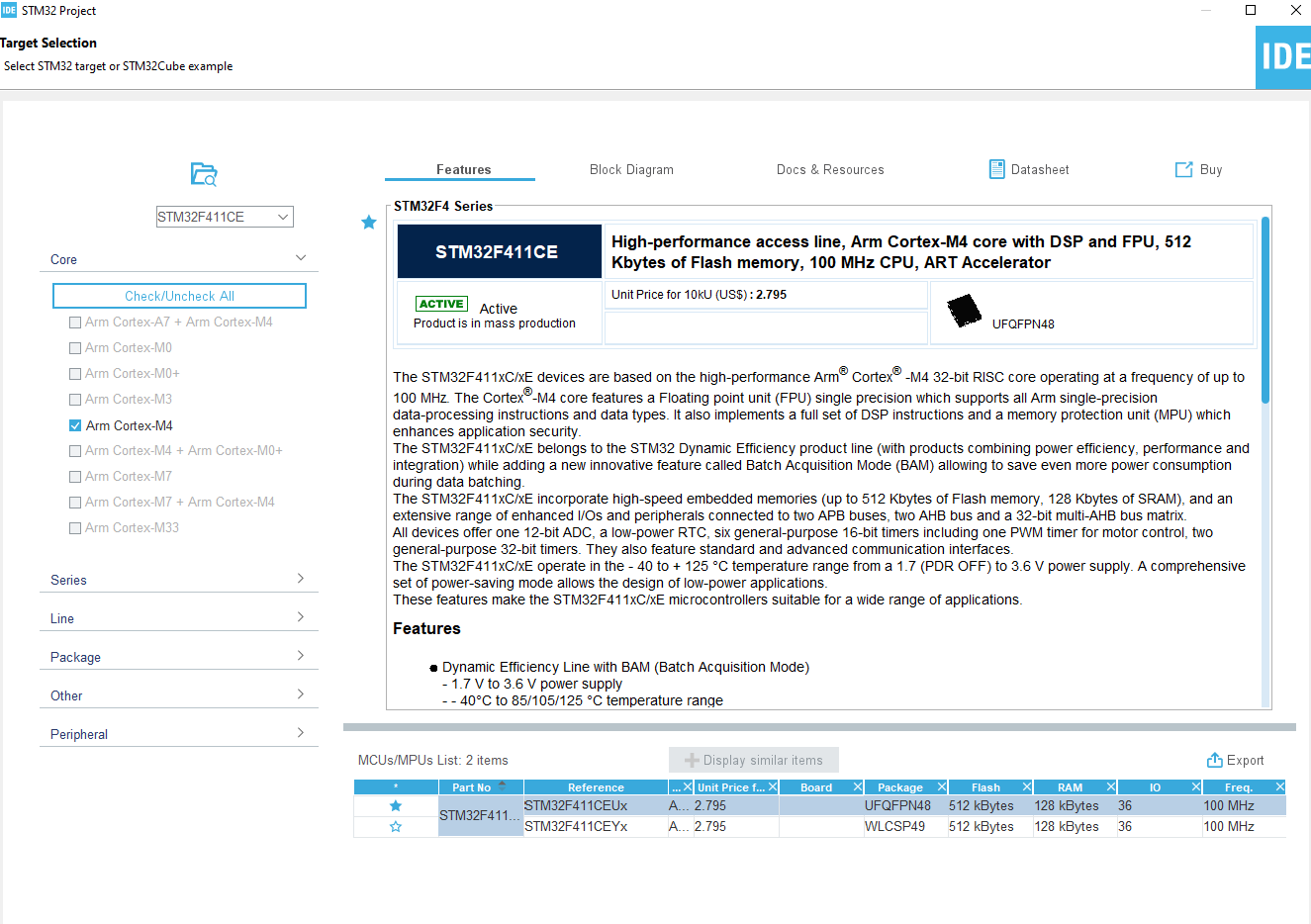This screenshot showcases an advanced network or computer management application, specifically geared towards managing STM32 microcontroller projects. The upper left corner features a small print header that reads "STM32 Project" accompanied by a blue logo with "IDE" in white text. Below this, users are presented with options for "Target Selection," which allows for the selection of an STM32 target or an STM32 Cube example.

The left column presents a structured menu for selecting specific components of the project, including options labeled "Core," "Series," "Line," "Package," "Other," and "Peripheral," each of which can be expanded to reveal further submenus. This organized hierarchy aids in navigating through various ARM Cortex cores and modules necessary for project customization.

Dominating the right side of the screen is a text box containing extensive technical details. A notable blue button with white text reading "STM32F411CE" is prominently displayed, indicating the selected microcontroller model. To the right of this button, there is bolded but small print terminology: "High-performance access line ARM Cortex M4, core with DSP and FPU, 512K bytes Flash memory, 100 MHz CPU, ART accelerator." An image of the chip is also visible, likely depicting the selected microcontroller.

The remainder of the text box is filled with intricate specifications and data, reflecting the depth of information available in the application. This detailed layout supports precise project setup and customization, crucial for professionals and enthusiasts working with STM32 microcontrollers.